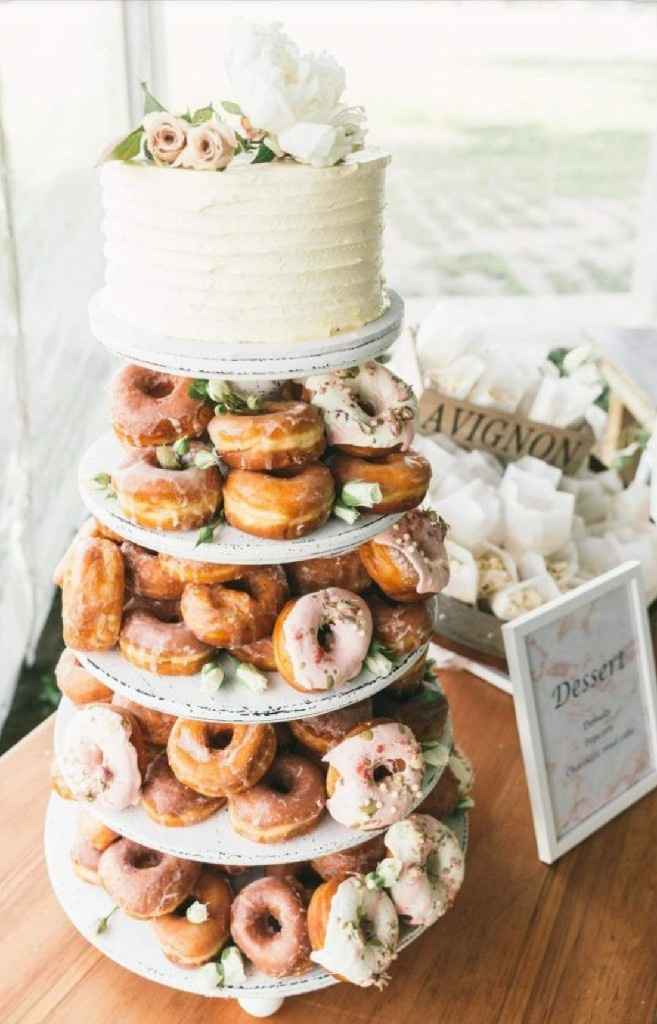The image captures a unique and elegantly arranged five-tiered dessert display, reminiscent of a traditional wedding cake stand but creatively adorned with beautifully decorated donuts instead of cake layers. Each tier of the stand is filled with a variety of donuts, some with dark icing, others with pink frosting adorned with white decorations. The top tier of this impressive display features a small white cake, garnished with an array of white and pink flowers, along with green leafy elements. Situated on a round table against a white background, possibly a wall or window, the display includes a sign labeled "Desserts" in black text on a white plaque. Another sign reads "Avignon" on a tan plaque amidst the flowers. The golden-brown donuts, some with white, pink, and green toppings, add a delightful contrast to the overall white-themed setup, making it a striking centerpiece for a celebratory occasion, likely a wedding.